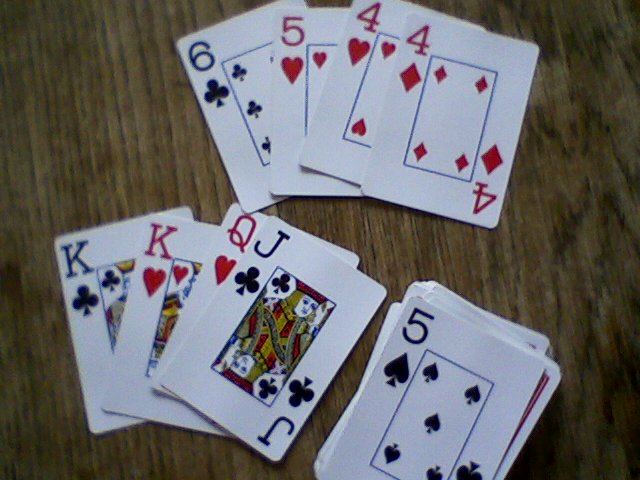This photograph showcases a traditional 52-card playing deck arranged on a wooden desk surface. The cards are notable for having slightly larger numbers and letters in the corners, thereby making the suits in the center a bit smaller than standard.

In the lower right corner, a five of spades card is prominently face up on top of a slightly staggered stack of face-down cards. The upper right corner of this stack reveals a glimpse of the card backs, which are red with a white border.

Two fan-shaped stacks of cards lie to the left of the five of spades. The first stack from left to right, bottom to top, consists of a king of clubs, king of hearts, queen of hearts, and jack of clubs. Directly above this configuration is another fan-shaped stack of four cards: from left to right, and bottom to top, a six of clubs, five of hearts, four of hearts, and four of diamonds.

The desk surface is a dull brown color, featuring a wood grain that runs vertically through the image. On the right side, the grain is slightly darker with wider streaks compared to the finer, lighter streaks on the left. The composition of the photograph draws attention to the contrast between the detailed cards and the textured wooden backdrop.